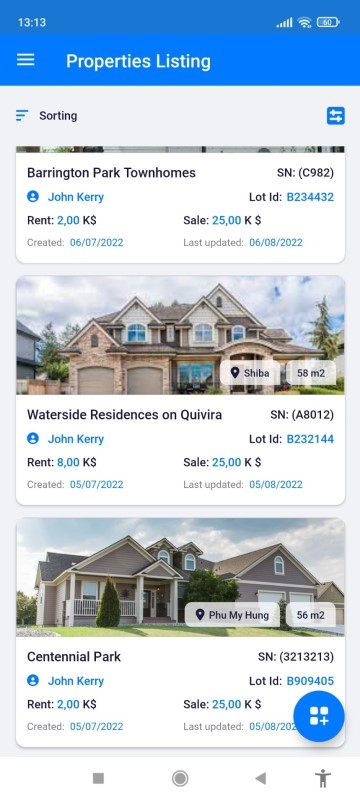This image is a screenshot from a cell phone displaying property listings. In the top right corner of the screen, the status bar shows a battery icon at 60%, a Wi-Fi symbol with three connection lines, and full bars of cell phone service. The upper left corner shows the time as 13:13. The top banner of the screen is blue with white text that reads "Property Listing." 

There are three property listings visible: 

1. **Barrington Park Townhouse**:
   - Listed by John Kerry
   - Rent: $2,000
   - Sale price: $25,000

2. **Waterside Residence on Quivira**:
   - Listed by John Kerry
   - Rent: $8,000
   - Sale price: $25,000
   - The image shows a large house with multiple front-facing windows, three peaked roof sections, and two separate garages.

3. **Centennial Park**:
   - Listed by John Kerry
   - Rent: $2,000
   - Sale price: $25,000